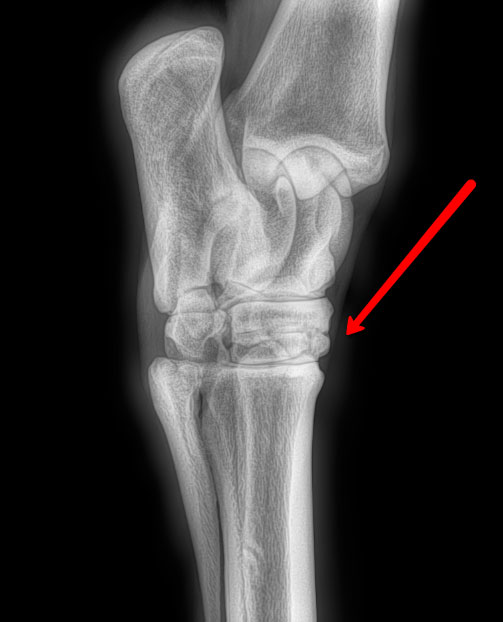This image is a detailed x-ray, featuring a complex joint that appears to belong to either a leg or an arm, possibly of an animal given the unusual structure. The background is completely black, sharply contrasting with the grayish-white bones. The x-ray reveals a straight bone at the bottom, connecting to a joint from which two additional bones extend. One of these bones does not join with the other, adding to the peculiar configuration. There is a distinct white halo around the bones. Moreover, a long red arrow is prominently pointing downward towards the middle joint area, possibly indicating a specific point of interest such as a break or fusion. The overall impression is one of intricate bone details standing starkly against a dark void.